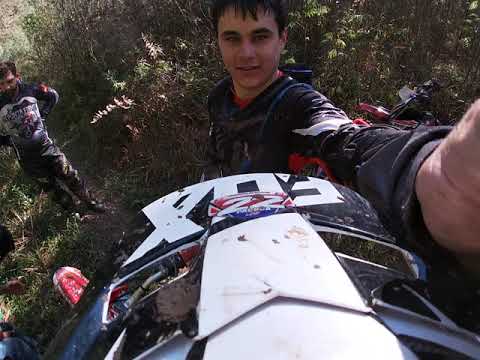The image captures two young men in a heavily wooded area, possibly hiking. The main focus is a close-up of a young man with short, brown hair, wearing a dark jacket with white accents. He seems to be taking a selfie, as he holds a camera pointed downward toward himself. In front of him is a black and white plastic object adorned with the number “22” in white on a red background, and the word "FOX" across the hood. This object, which may resemble a toy car or a machine part, has a shiny, metallic appearance with what look like windows or vents on its sides. To the left, another young man with brown hair, sporting a mustache and beard, is partially visible. He is also dressed in a dark long-sleeved shirt with a white design and pants. Both men have some red attachments on their arms, possibly pieces of equipment. The background reveals a mix of brown earth, green patches, and branches, emphasizing the outdoor, wooded setting.